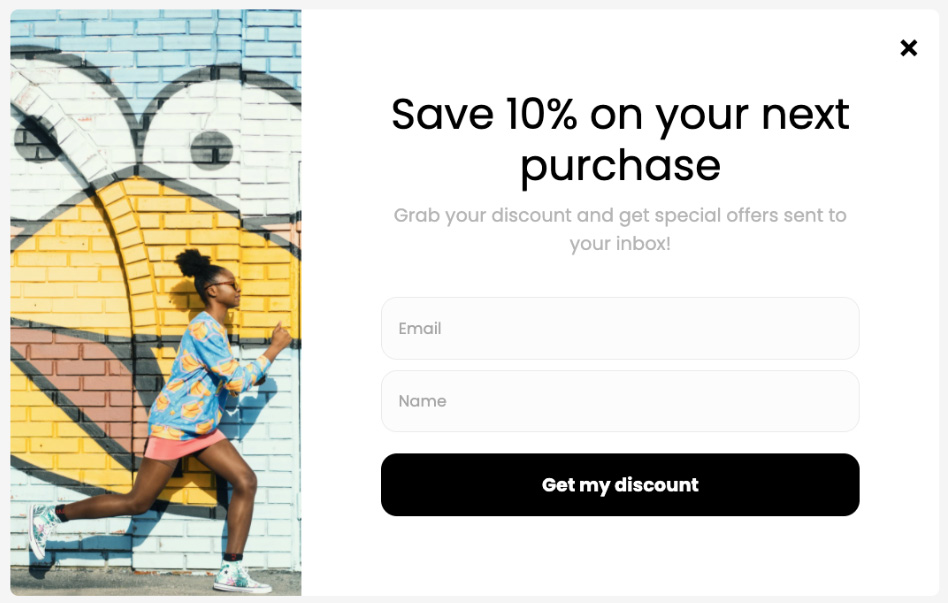The image captures an urban scene featuring a vibrant street art mural on a brick wall. The mural depicts a stylized bird face, meticulously crafted with bold and vivid colors. The top portion of the wall is composed of blue bricks, setting a contrast for the bird's eyes. The eyes are large, outlined in black, and filled with solid black pupils that stand out against the background. The beak of the bird is strikingly orange, bordered with black, and features a red interior that adds depth and intrigue to the artwork.

In the foreground, an African-American girl can be seen running past the mural. Her hair is styled in a high ponytail, and she dons a pair of glasses. She wears a blue shirt adorned with a playful banana print, paired with a skirt, which emphasizes her lively movement in the urban environment.

To the right of the image, a promotional box offers a discount, stating, "Save 10% on your next purchase. Grab your discount and get special offers sent to your inbox." It includes fields to enter an email and name, accompanied by a prominent black button labeled "Get My Discount." This visually appealing composition combines street art and commercial elements, capturing the dynamic essence of city life.